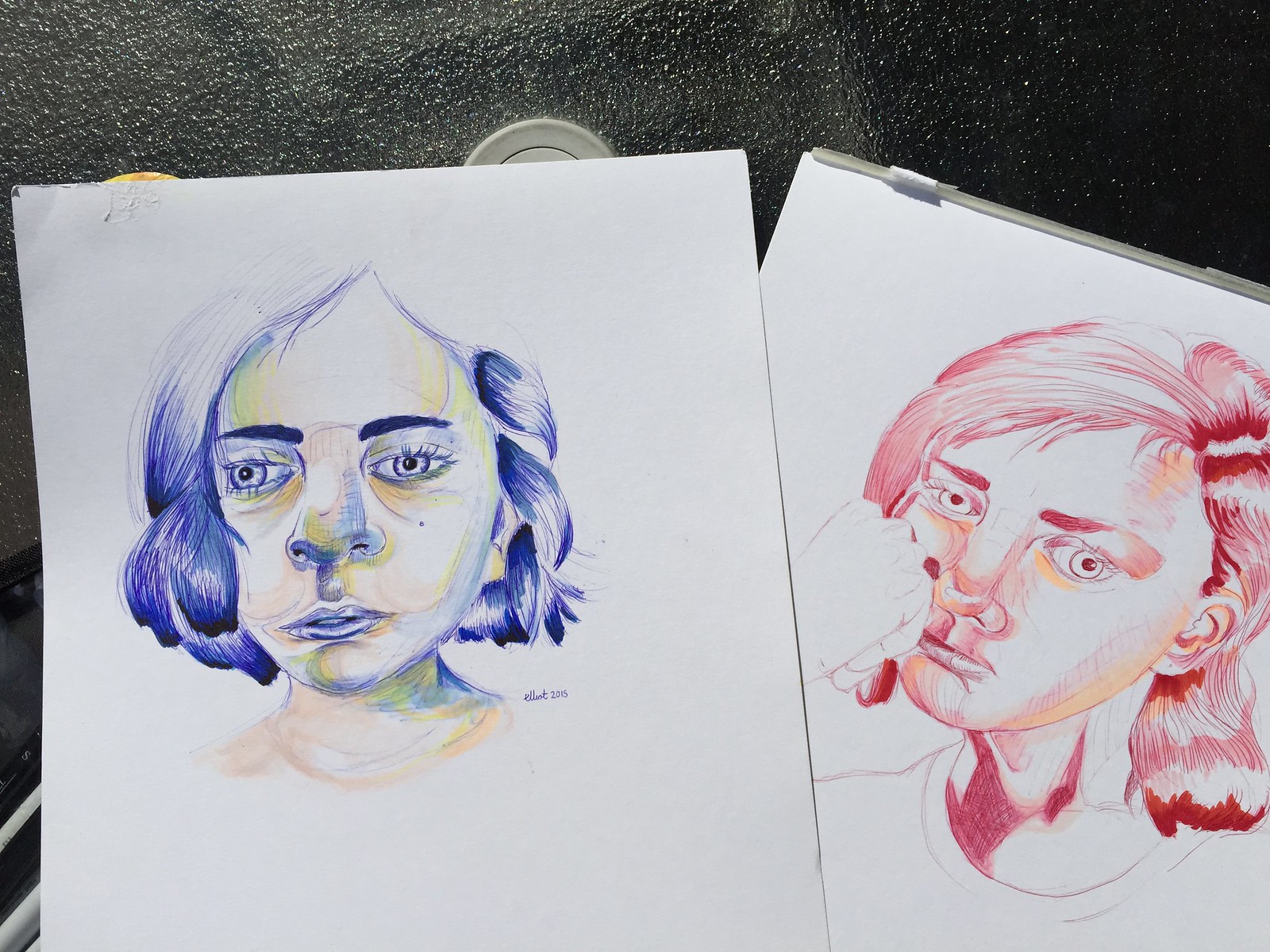This captivating image showcases two distinct pieces of art, each drawn on a separate sheet of white paper, both placed on what seems to be a speckled black countertop, possibly granite. The top-left sheet features a vibrant portrait of a young girl, illustrated with a vivid palette of blues, greens, peaches, and yellows. Her hair and eyes are prominently blue, while the outlines and other facial details are skillfully accented with touches of green, yellow, and peach. The artistry highlights her delicate features with a blend of cool and warm tones that bring her expression to life.

Beneath this first drawing, on the right side of the image, lies another portrait, created in a similar expressive style. This second girl is depicted using a rich spectrum of reds and oranges, lending a warm, fiery intensity to the piece. Her hair, imbued with various shades of red, cascades down as she thoughtfully rests her chin on her balled-up fist. The dynamic use of warm colors exudes a sense of deep contemplation and emotion, contrasting beautifully with the cooler hues of the portrait above.

Overall, the image captures the engaging contrast between the two expressive portraits, set against the striking, speckled black surface, enhancing their vividness and the emotions they convey.